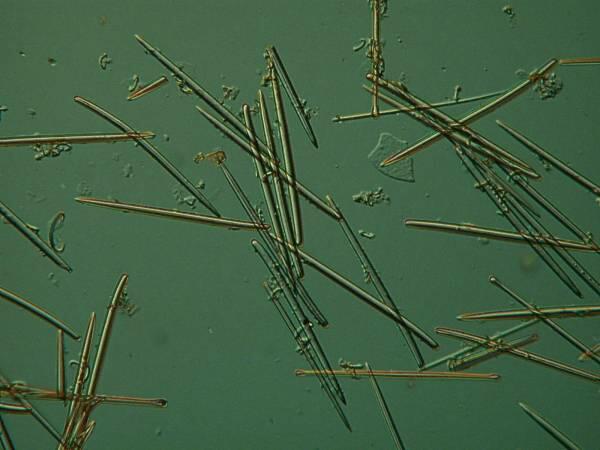The image depicts a highly magnified view, likely captured through a microscope, of numerous elongated, needle-like structures scattered across a dark green-gray or navy-green background. These rod-like formations, some of which exhibit a yellowish tinge while others blend into the same hue as the background, appear to be arranged haphazardly and without any discernible pattern. The translucent structures resemble toothpicks or crystals in a fluid, seemingly piled unevenly atop one another. Despite the close-up perspective that suggests a microscopic slide, the image lacks any descriptive text or context, and it is cropped, offering only a partial glimpse of the overall scene.